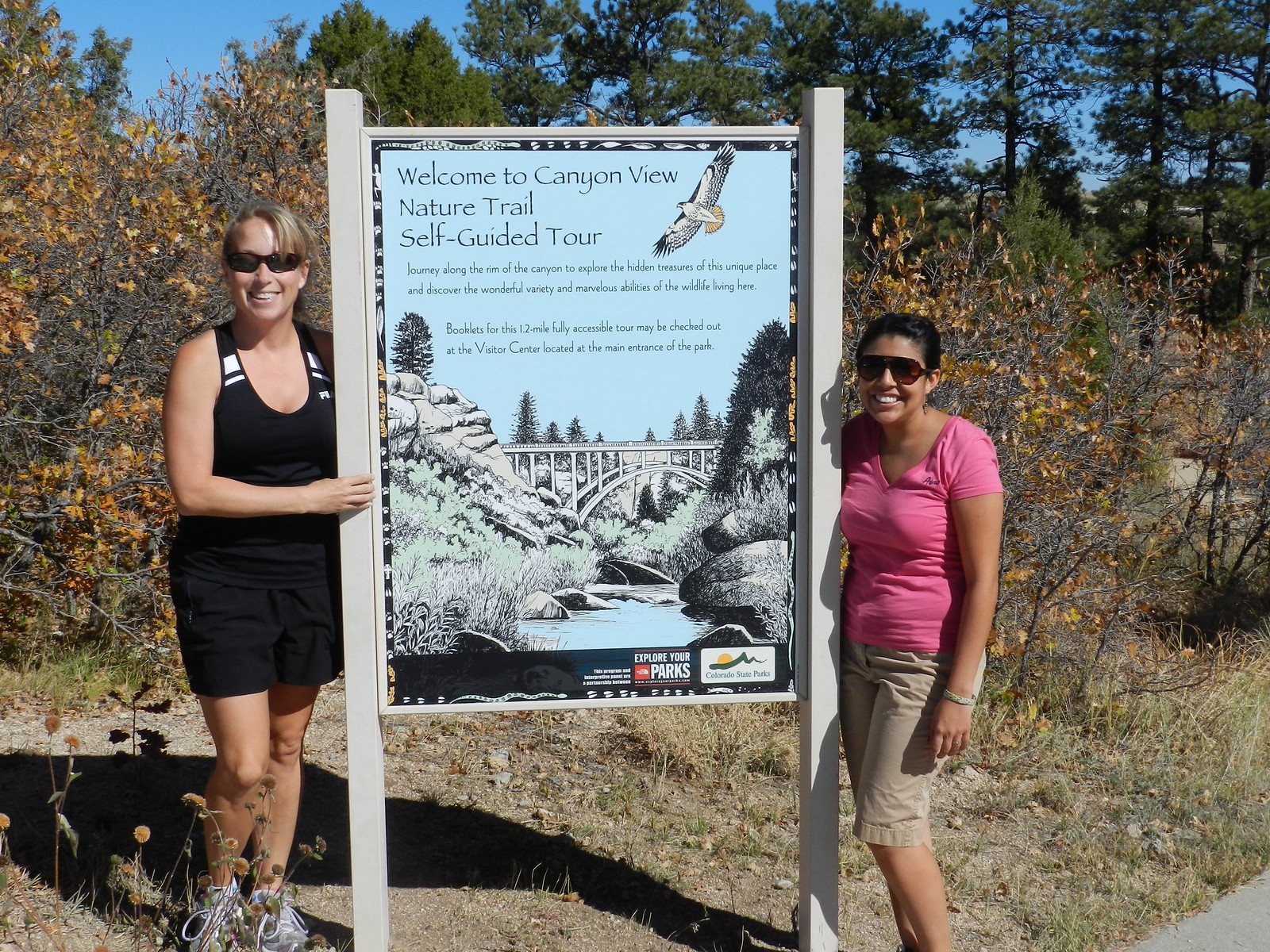The image depicts two women standing outdoors on what appears to be a bright, sunny day, against a backdrop of pine trees and shrubs with dead or brown leaves, suggesting an autumn setting. Both women are wearing sunglasses, and there's a prominent sign between them. The woman on the left is Caucasian, with light brown hair and dark glasses, dressed in a black tank top with yellow highlights on the sides, black shorts, and tennis shoes partially obscured by branches. The woman on the right, who appears to have a Hispanic heritage, has dark hair and is wearing a pink t-shirt with khaki shorts, smiling warmly. The sign between them reads, "Welcome to Canyon View Nature Trail — Self-Guided Tour," and features an illustration of a bird, likely an eagle or hawk, along with images of a creek, a bridge, rock hills, and more greenery. In the background, the sky is visible above the trees and lifeless shrubs, completing the scenic outdoor setting of the nature trail.